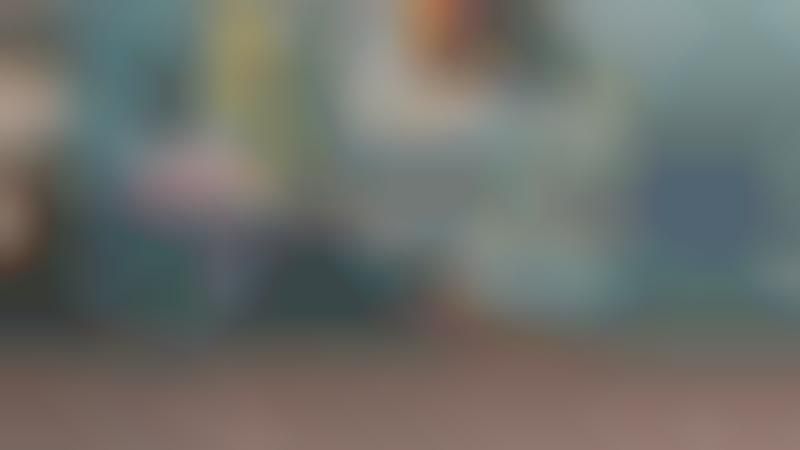In this image, a brown and white dog is lying down on a brown wooden boardwalk or deck. The dog has white on its face, chest, and paws, and wears a blue collar attached to a green leash with a yellow end. It holds a yellow tennis ball in its mouth with black text on it. The dog’s front paws are extended forward, its head is slightly turned to the right, and its back legs are angled to the right. 

Behind the dog is a detailed mural featuring a woman holding up a trophy with the text "Champion 2016 Osaka" prominently displayed. The mural showcases various elements including repeated words "deuce" and "advantage," with a mix of blue, gold, white, and pink colors. In the bottom right corner of the mural, the text "ESPN" can be seen along with a cut-out of "New York". 

To the left of the dog, a woman is leaning against the wall. She has black-framed sunglasses with silver ear pieces, and is dressed in a black t-shirt and blue jeans. She is also wearing earrings. Behind her, a white building with silver bars on the windows and a silver pole is visible. The mural includes a city landscape on the right side with mostly blue buildings that have yellow tops and light blue accents.